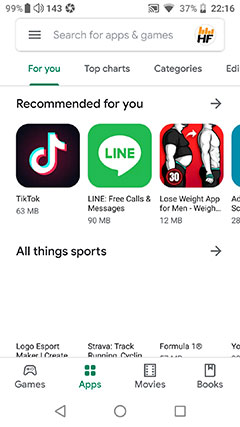The screenshot displays the Google Play Store interface on an Android mobile phone, identifiable by the navigation bar at the bottom which includes three icons: a left-pointing arrow for "Back," a circle for the "Home" button, and a square for "Recent Apps." The image features a light background typical of the Google Play Store. 

At the very top, a search bar with a light gray outline is visible, allowing users to input queries. Below the search bar, several clickable text-based tabs are present. These include "For You," "Top Charts," and "Categories." The "For You" tab is highlighted in green, indicating it is currently selected, while the other tabs remain in black.

Further down, there is a "Recommended For You" section displaying app suggestions. Visible in this row are the TikTok app, characterized by its black square icon with a musical note inside, and the Lion app, distinguished by its green icon with a speech bubble.